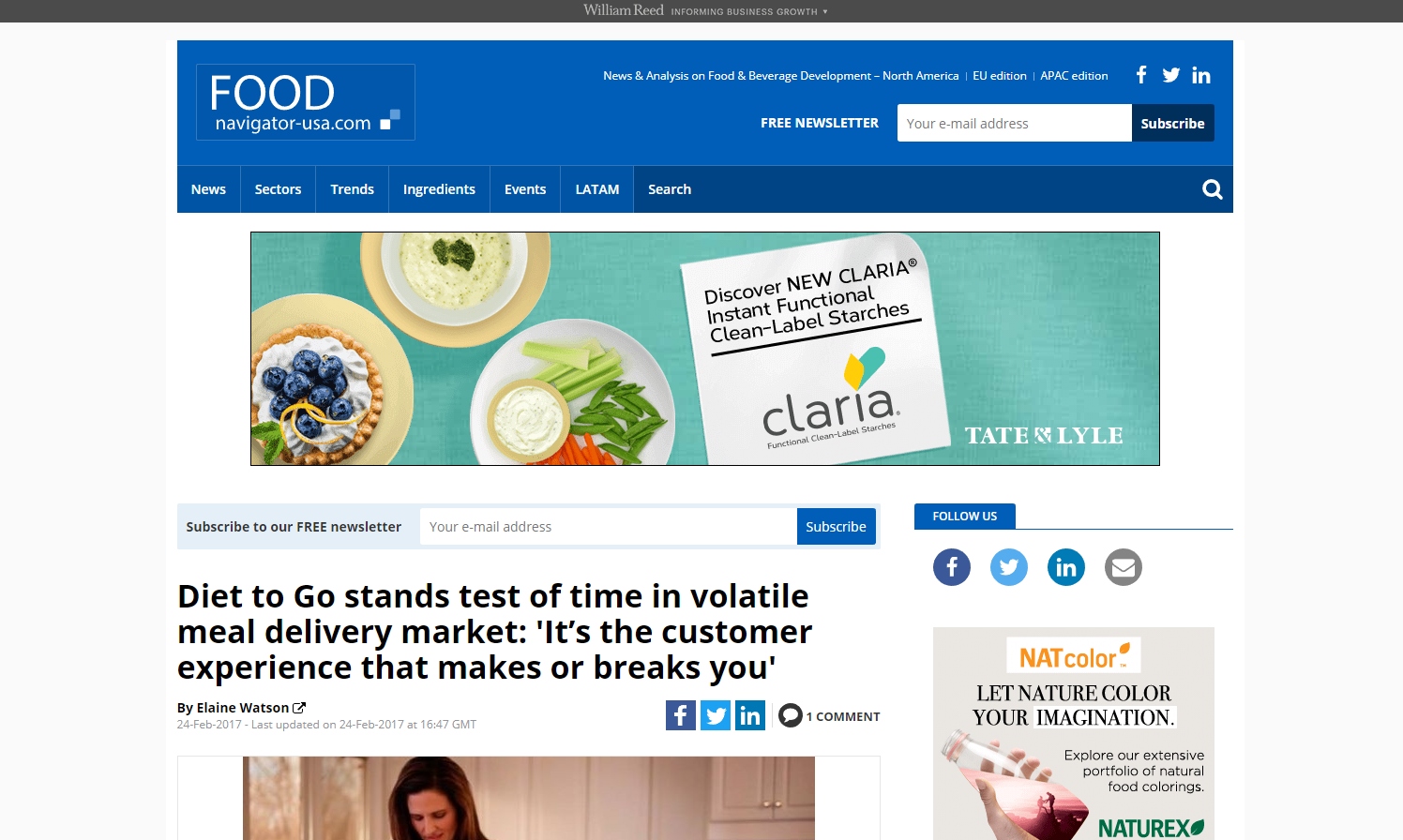This screenshot captures a detailed view of a web page from FoodNavigator-USA.com.

The thin gray header bar at the top prominently features small-centered text reading "William Reed: Informing Business Growth" with a downward arrow. The main header of the web page, which is slightly indented on both sides, displays the FoodNavigator-USA.com logo in the upper left corner. A navigation bar runs across the top, including categories such as News, Sectors, Trends, Ingredients, Events, and LATAM, alongside a vibrant blue search bar. Adjacent to this navigation bar are three social media icons and a section to sign up for a free newsletter, requiring just an email address to subscribe.

Beneath the header, an ad banner showcases a vibrant photograph of three plates of food with the text "Clarillo, Taste or Tate and Lyle." Directly below this is a subscription button for the free newsletter, followed by an engaging article titled "Diet To Go Stands Test of Time in Volatile Meal Delivery Market. It's the Customer Experience That Makes or Breaks You." The article is attributed to its author, whose name and a cropped photo of a woman's head appear alongside additional icons.

To the right of the article, there is a "Follow Us" section featuring icons for Facebook, Twitter, LinkedIn, and email. At the lower right-hand corner of the page, an advertisement for Naturex is displayed, featuring a photograph of a woman's hand holding a glass bottle with an image inside it. The overall layout is designed to provide readers with an immersive and user-friendly experience.